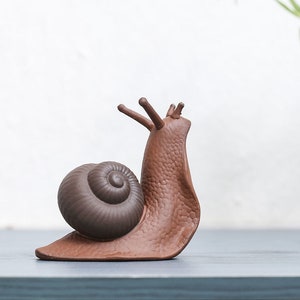This photograph features a detailed figurine of a snail or slug with a shell, placed on a smooth, blue-stained wooden surface. The figurine’s body is a warm reddish-brown color, resembling terracotta, while the shell is a darker, chocolate brown with a swirling pattern that narrows to a central point. The snail is depicted with its body partially lifted off the surface, giving the impression that it is gazing upward. Its antennae and eyes are prominently extended, contributing to its lifelike appearance. The background of the image is brightly lit and predominantly white, with a slight blur and a hint of greenery visible in the upper right corner. Despite the snail's realistic features, the proportions suggest it is an artistic, clay or plastic model rather than a real creature.